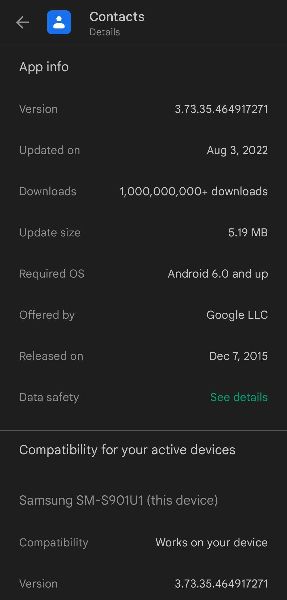The image is a detailed screenshot of the Contacts app information page. At the top center, the header reads "Contacts," with a subheading underneath labeled "Details." To the left, it displays "App Info." The specific version of the app is listed as 3.73.35.46.49.17.2071, showing it was updated on August 3rd, 2022. The app has amassed over 1 billion downloads, with the most recent update size being 5.19 MB. It requires an operating system of Android 6.0 or higher to function. The app is offered by Google LLC and was initially released on December 7th, 2015. For data safety information, there is a green prompt stating "See details."

The next section addresses compatibility with active devices, specifically mentioning the Samsung SM-S901U1, which is confirmed to be the current device. It states, "Compatibility works on your device," and reiterates the version number 3.73.35.46.49.17.2071. The overall background of the image is a dark grey.